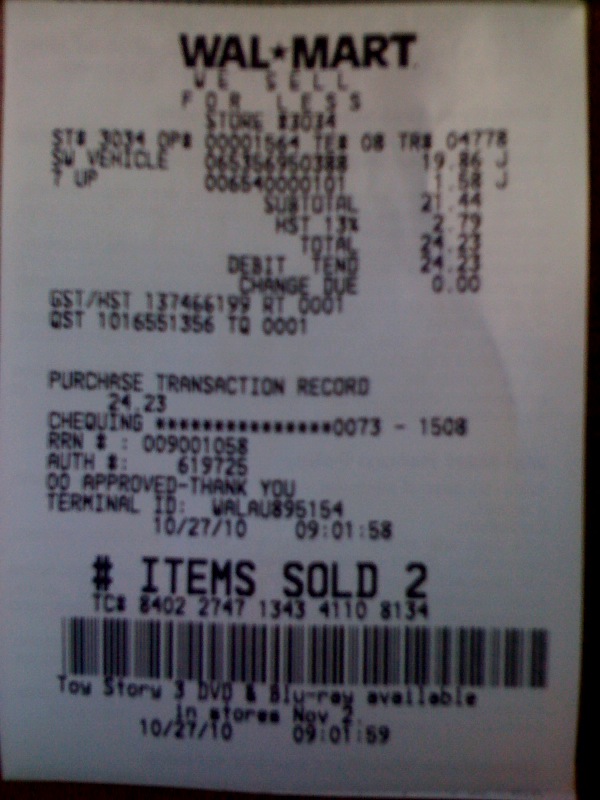The image showcases a detailed Walmart receipt from October 27th, 2010, at 9:01:59 AM from store number 3034. The receipt, printed in black ink on white paper, prominently displays the store's slogan, "Walmart - We Sell for Less," at the top. The transaction totaled $24.23, paid via a checking account. The receipt denotes that two items were sold, and beneath the barcode at the bottom, it has a promotional message: "Toy Story 3 DVD and Blu-ray available in stores November 2." It also includes approval details and a terminal ID, with a purchase transaction number 1508 documented.